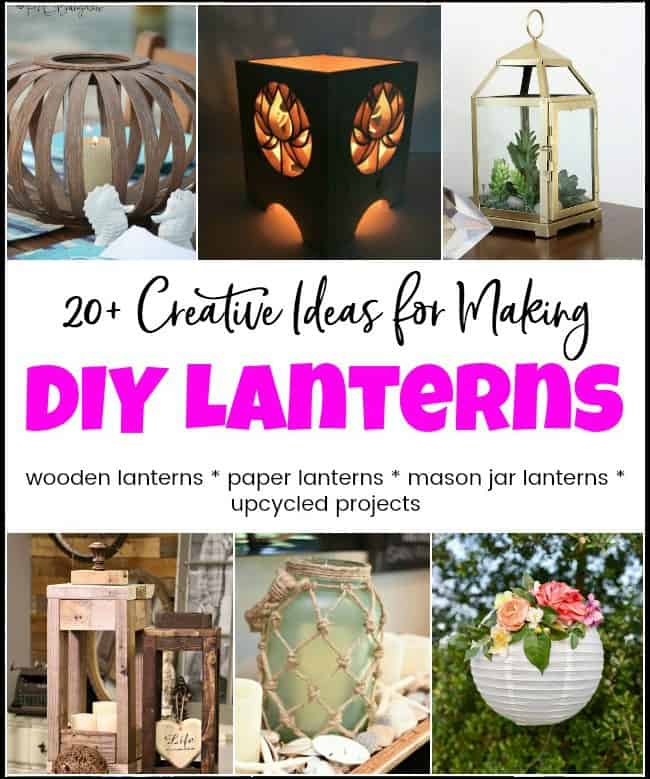This image is the cover of a book titled "20+ Creative Ideas for Making DIY Lanterns," featuring a white horizontal bar at the center with text. The title is presented with "20+ Creative Ideas for Making" in a cursive black font, while "DIY Lanterns" is emphasized in bold pink (or purple) font. Below the main title, there is a list of lantern types included in the book: wooden lanterns, paper lanterns, mason jar lanterns, and upcycled projects.

The cover is adorned with a grid of six small photos, three at the top and three at the bottom. In the upper row, from left to right:
1. A bamboo-style wooden lantern with a candle inside, spherical in shape reminiscent of a tomato.
2. A black lantern with intricate designs and orange lighting creating a box-like appearance.
3. A gold lantern shaped like a light fixture, creatively holding green plants inside.

In the lower row, from left to right:
1. A wooden lantern, possibly rustic in design, also with lit candles inside.
2. A mason jar lantern adorned with macrame, providing a stylish lighting solution.
3. A white paper lantern designed with decorative flowers, appearing collapsible like a sphere.

Each image offers a glimpse into the diverse and imaginative lantern projects detailed in the book.